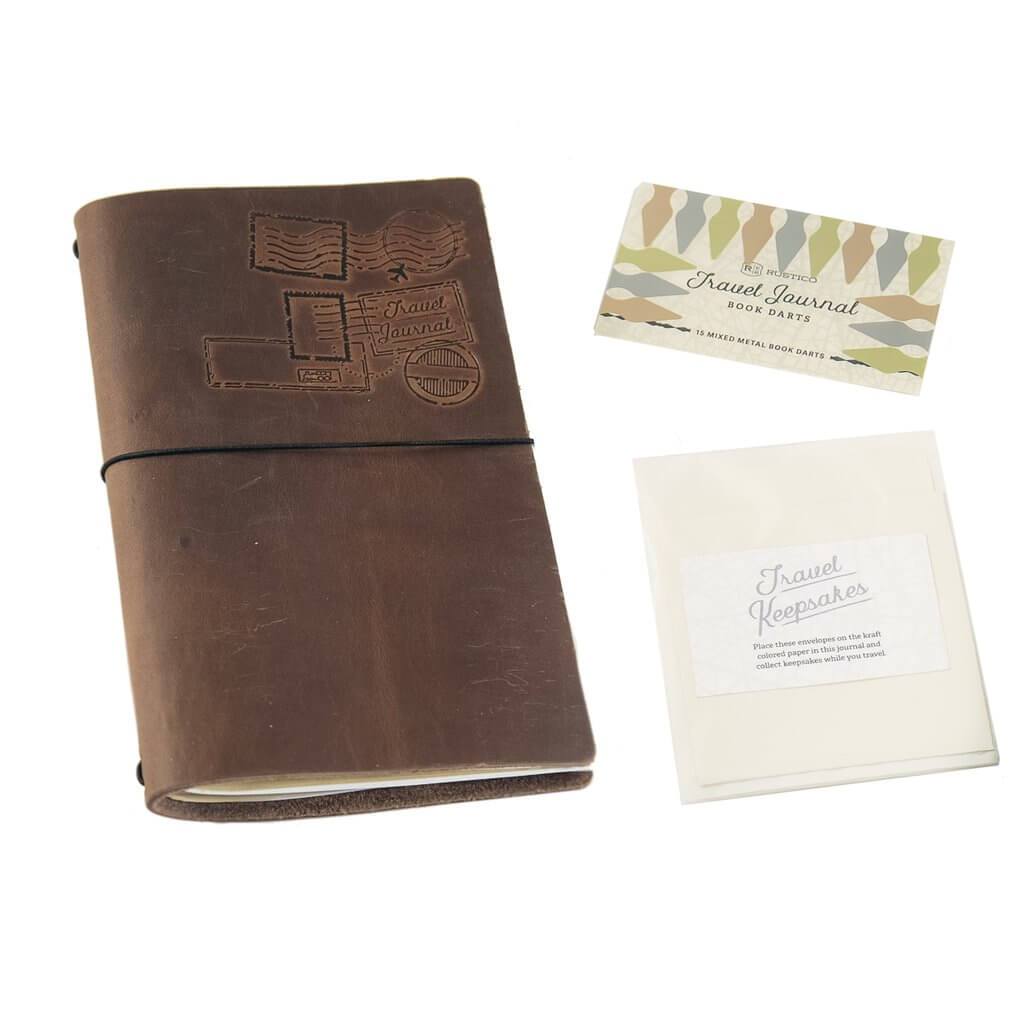The vertical image showcases a well-worn, brown leather-bound notebook, resembling an old journal or dress book, with imprinted and embossed stamps, including a tiny airplane and the words "Travel Journal." The notebook is fastened shut with a fancy black band. To the top right of the journal, there is a note card labeled "Rubsico Travel Journal Book Darts, 15 mixed metal book darts," surrounded by pastel-colored fountain pen tips or darts meant for bookmarking. Below this card, there is a plain white envelope or pouch labeled "Travel Keepsakes," with additional small, unreadable text.